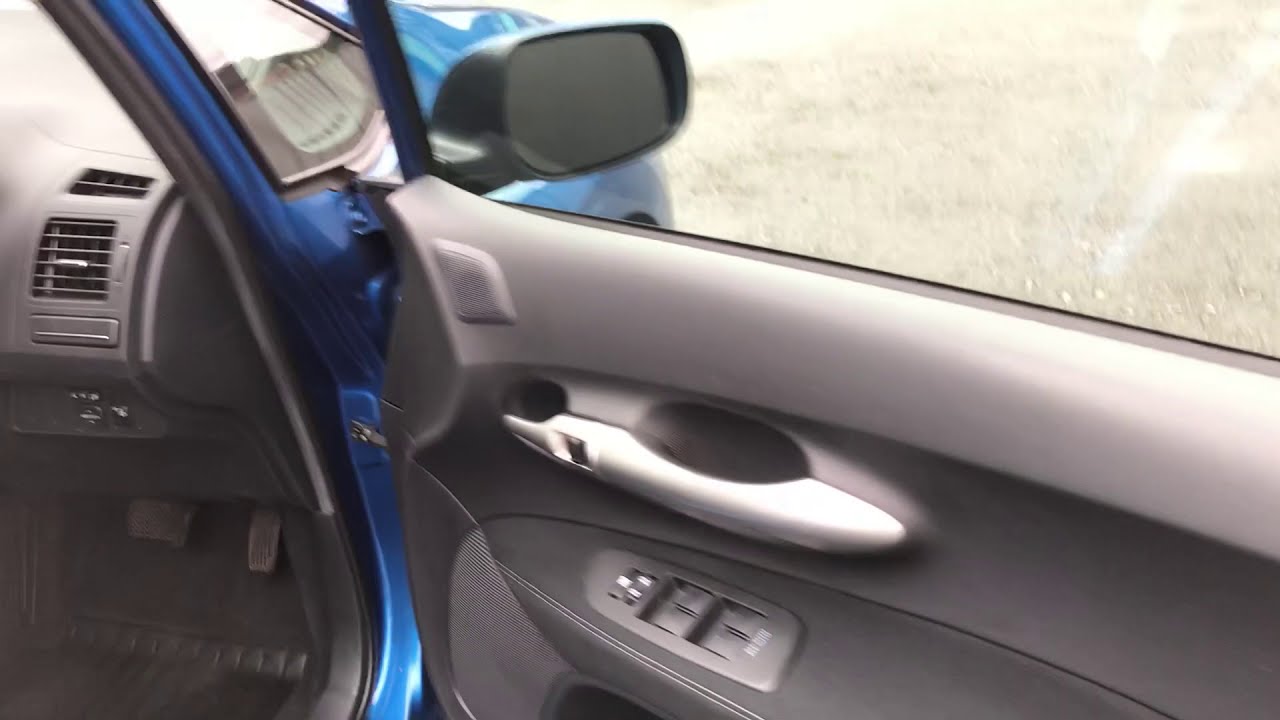This image showcases the interior of a modern car with a shiny metallic blue exterior. The photo predominantly focuses on the right side of the car's interior, which is likely a foreign model considering the positioning of the pedals on the right. The car door, which is a combination of gray and silver hues, is prominently featured with an inner door handle and a set of square electronic buttons, possibly for window operation. Above the pedals, an air conditioning vent can be seen. The photo is taken during the daytime, evidenced by the clear view through the window which reveals some pavement outside and the passenger side mirror. Additionally, the blue exterior of the car is clearly visible through the window. The interior also exhibits hints of beige and brown tan colors, contributing to the sleek look of the modern vehicle.